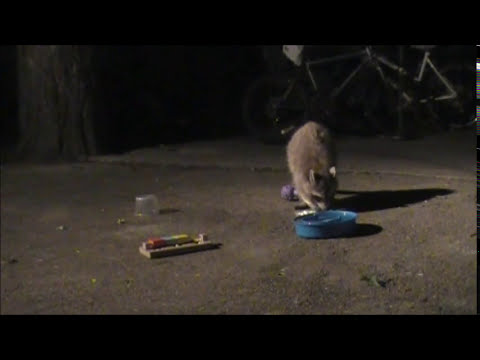The image depicts a nighttime outdoor scene of a grainy, low-quality photograph dominated by digital artifacts and splashes of yellow noise. The main focus is a classic brown raccoon with distinctive black markings around its eyes, positioned slightly to the right of the center. The raccoon is hunched over a blue bowl, seemingly attempting to eat from it or playing with it, using its paw to pull the bowl closer. 

The ground beneath the raccoon is a cement pavement littered with various objects, including some pieces of trash and a clear bowl. To the left of the raccoon, there's a piece of wood with a multicolored stick, possibly resembling a rudimentary trap. The background features a large tree and some bicycles with white frames parked against a pole, and hints of graffiti on a wall. The entire scene is illuminated with dim lighting suggestive of a dark alley devoid of human activity, with the raccoon being the central element of this nocturnal setting.